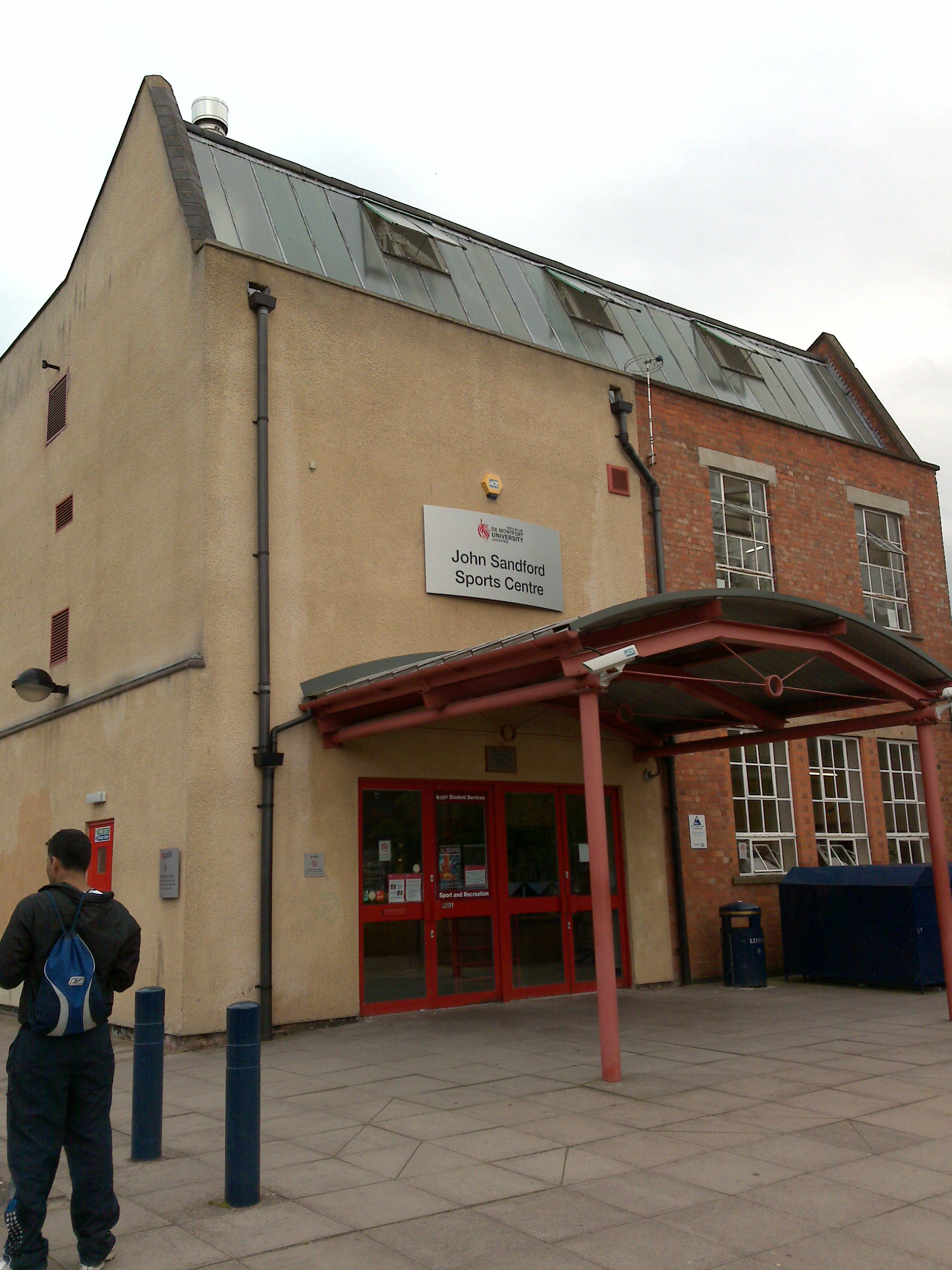The image depicts a tall building with distinct architectural features. The structure is split into two contrasting sections: one half is covered in a tannish-yellow cement, while the other half showcases reddish brick. The brick side features two upstairs windows and three downstairs windows, all with white grids. A prominent arched porch marks the entrance, supported by metallic rafters and two metal front legs. The building entrance includes four doors with red frames. Above the entrance, signage reads "John Sanford Sports Centre," accompanied by a logo for "Dumontford University," and a yellow hexagonal ADT alarm is affixed to the wall. The exterior ground is paved with cement square lines. In the scene, a man dressed in an all-blue outfit and wearing a backpack stands to the side of the building. The sky above is cloudy but bright, adding a contrasting backdrop to the vivid architectural details.